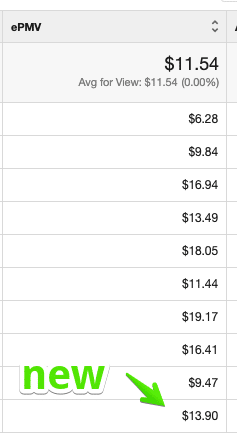This screenshot features a predominantly white background dominated by a vertical, slightly gray rectangular drop-down menu located at the top. The drop-down menu is labeled "EPMV," with a lowercase 'E' and uppercase 'PMV' in a bold black font. In the top-right corner of this menu, there are up and down arrows for navigation. Below the "EPMV" label, the number "1154" is prominently displayed in bold. Further down, it notes "average for view 11.5400%."

Below this header, a list of numbers is presented, each separated by thin, light gray lines. The numbers listed sequentially are: 628, 984, 1694, 1349, 1805, 1144, 1917, 1641, 947, and 1391. The numbers are also in a bold black font against the white background.

In a larger, lime green font, the word "NEW" is positioned prominently, accompanied by a downward-pointing arrow aimed at the number 1391, indicating it as the most recent entry. Beneath the "NEW" label, a wave-like design provides a subtle visual element. Overall, the screenshot is highly symmetrical, structured, and easily navigable.